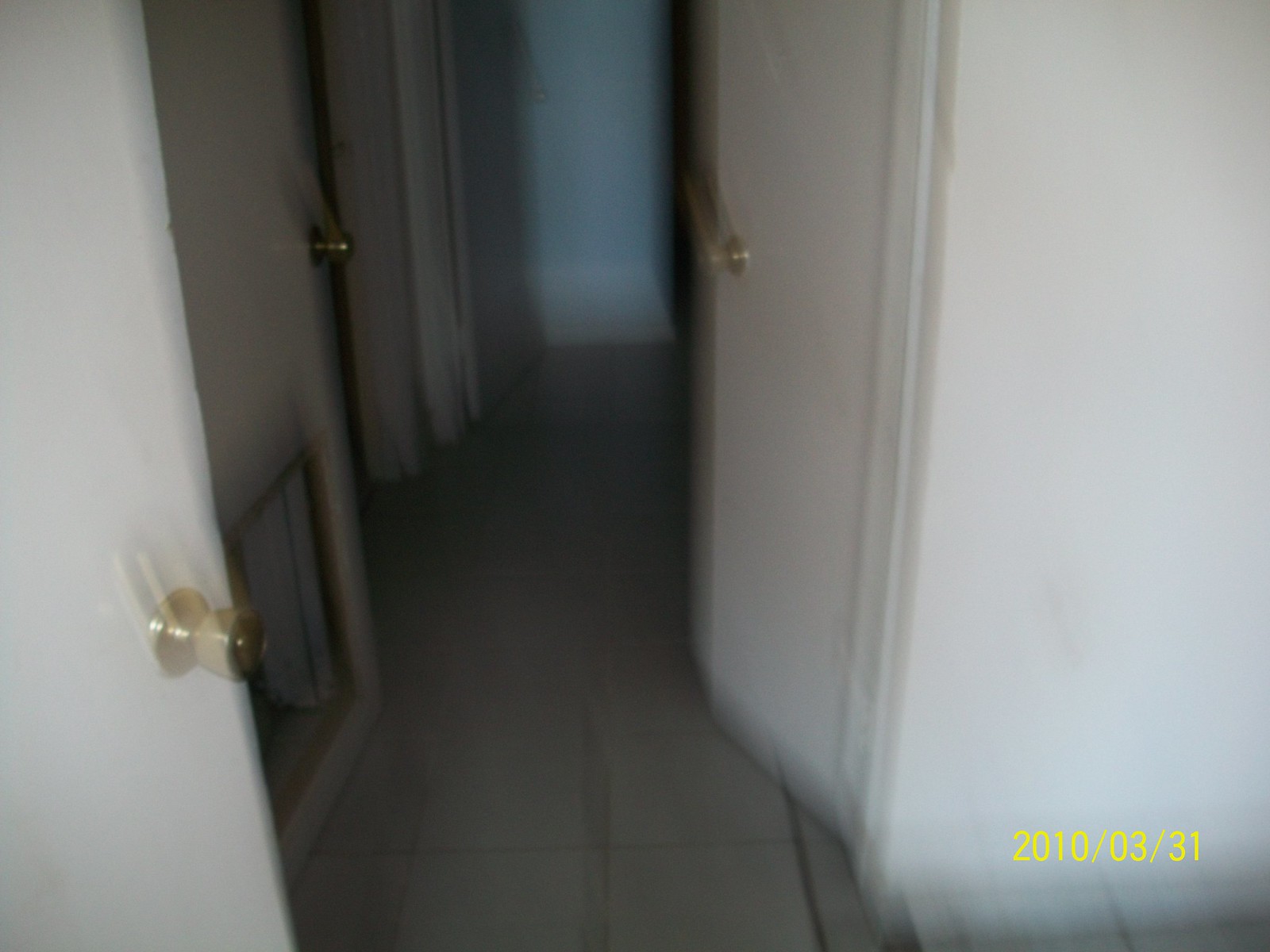This blurry image captures a hallway in a standard home, dated March 31, 2010, displayed in yellow text at the bottom right corner. The white walls and large white tiled flooring characterize the hallway. Three doors with gold doorknobs are visible: the closest door on the left is slightly open, another farther down the hallway on the left is closed, and a third door on the right is also ajar, allowing some light to spill into the hall. Notably, the door farther down the hallway on the left features a small gold doggy door at the bottom. The overall blur suggests the photographer was in motion while taking the picture.